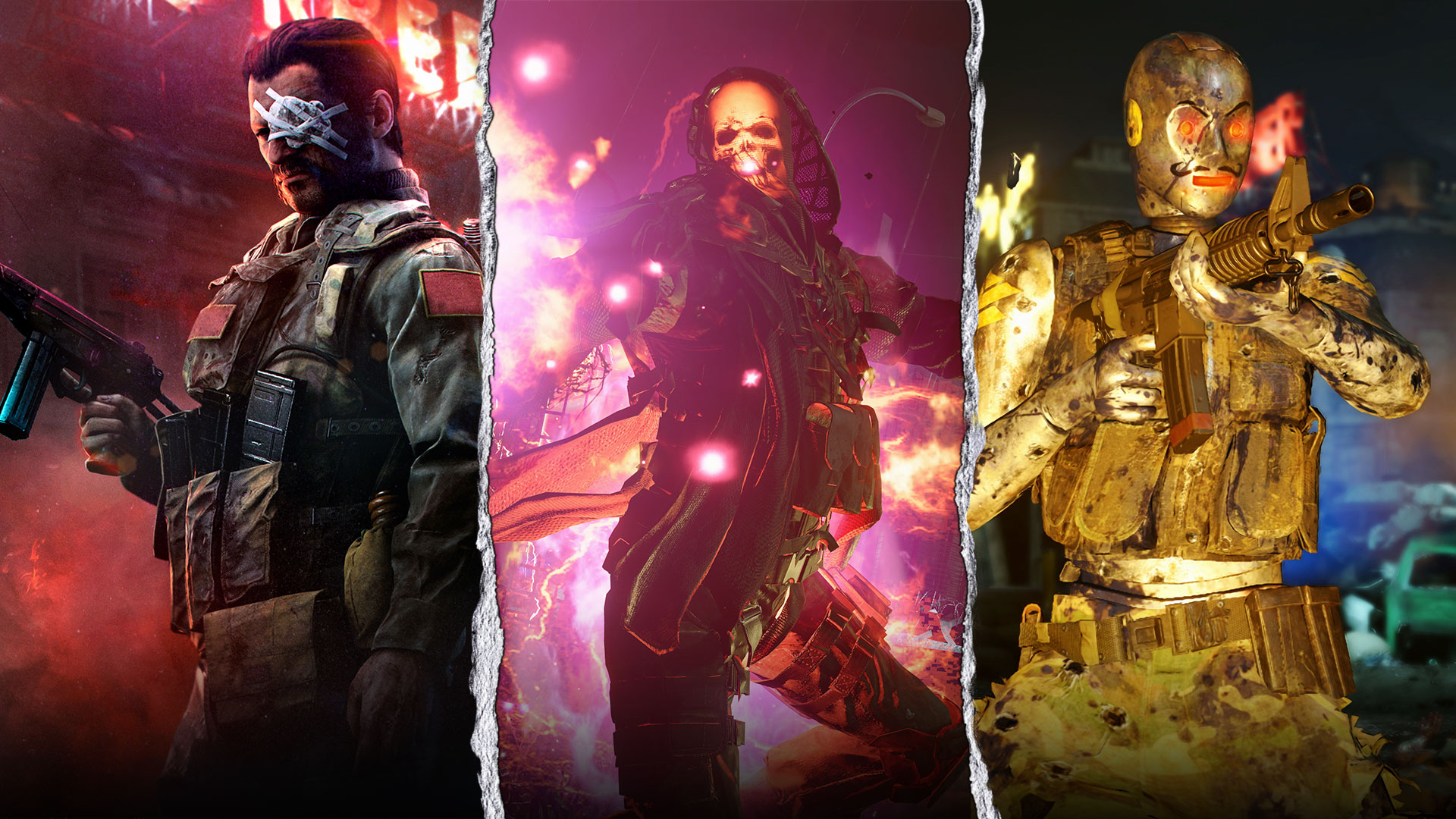This image appears to be an illustration or screenshot from a video game, featuring three distinct characters standing side by side, each with their own unique setting and aesthetic. 

On the left, there's a man with slicked-back hair dressed in a military uniform. He's holding a black machine gun in his right hand. His left eye is covered with a white patch secured by white tape crisscrossing over it. He sports a very short cut mustache and beard. The background behind him is red-hued and includes a lit street sign and a building partially obscured by fog.

The middle character is shrouded in a black hood and attire, which seems to be a mesh or net hood. His face resembles a glowing golden skull. The background is filled with vibrant purple and pink hues, elements of fire, and apparent fireworks, adding to the eerie and intense atmosphere.

On the right, the character resembles a golden cyborg, evoking visual similarities to C-3PO. This character is armed with a machine gun, which appears to be actively firing. The eyes and mouth are glowing red, and there is visible dark environment behind, along with a car partially visible in the shadows. 

Each character's design and background contribute to an overall theme of high-intensity, possibly combat-oriented, scenes reflective of video game fantasy or science fiction genres.